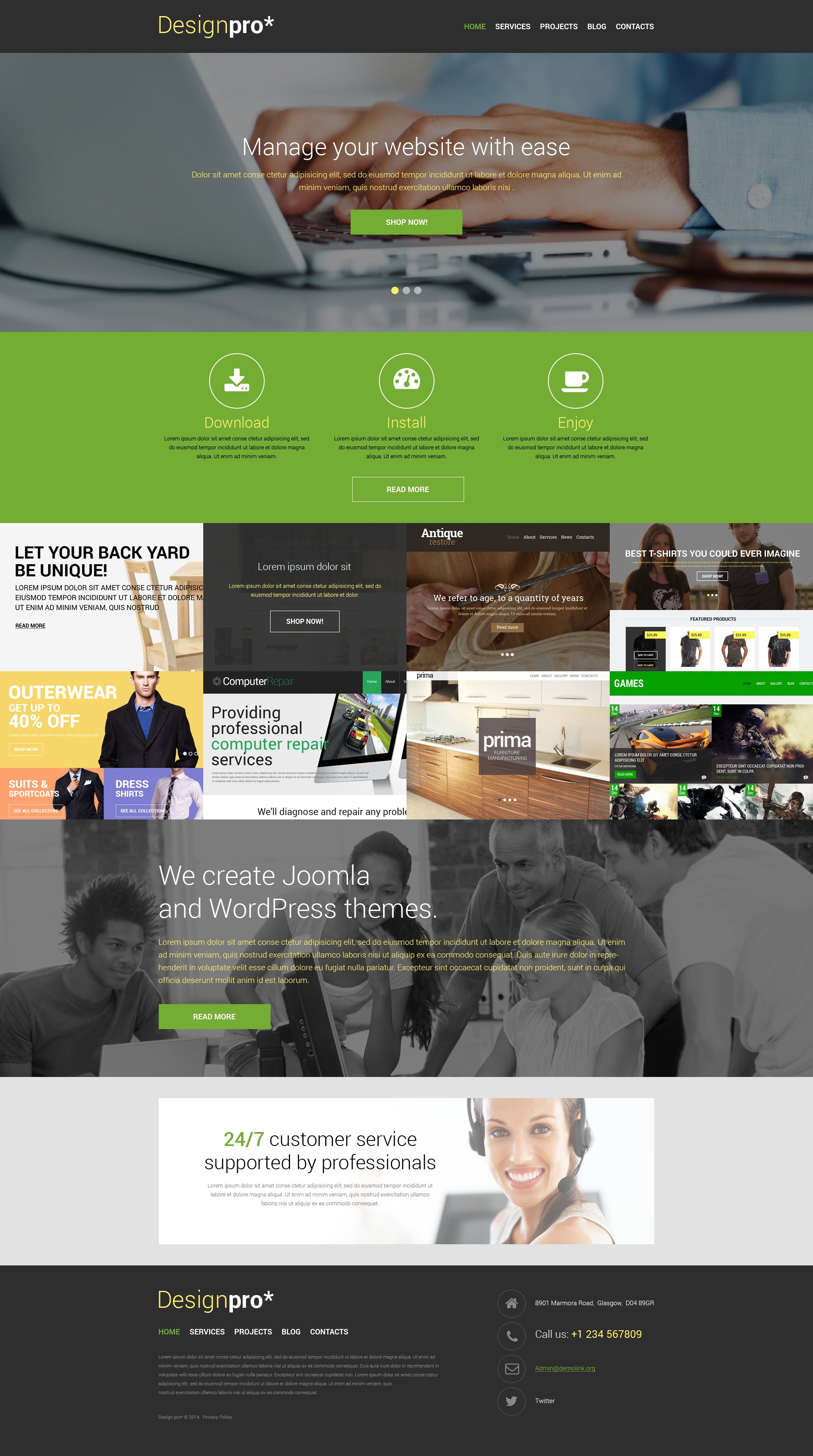This image is a promotional banner from the website "Design Pro," prominently displayed at the top in a black bar with "Pro" highlighted in a slightly brighter white than "Design." The main tagline beneath this header reads, "Manage your website with ease," accompanied by a green "Start" button centrally located. Below the tagline, there is a photograph of hands typing on a laptop keyboard, suggesting the ease of managing a website using Design Pro's tools.

Further down, the banner showcases various advertisements for different products. One of the ads highlights a man wearing a jacket, promoting "Court Outerwear" at 40% off. Another advertisement features "Prima," while another offers "Professional Computer Services." Each ad is distinct, catering to a variety of products and services.

Following this section is a gray area stating, "We create Zoomia and WordPress themes," depicting a diverse group of people gathered around a computer, symbolizing teamwork and inclusion. Directly below this is a lighter gray section with a white rectangular box containing the message, "24-7 customer service supported by professionals," next to an image of a smiling woman wearing headphones, indicating friendly and continuous customer support.

At the very bottom, another black bar displays "Design Pro" alongside contact information, with the phone number notably highlighted in yellow for easy visibility. This comprehensive layout effectively conveys the various services and features offered by Design Pro.